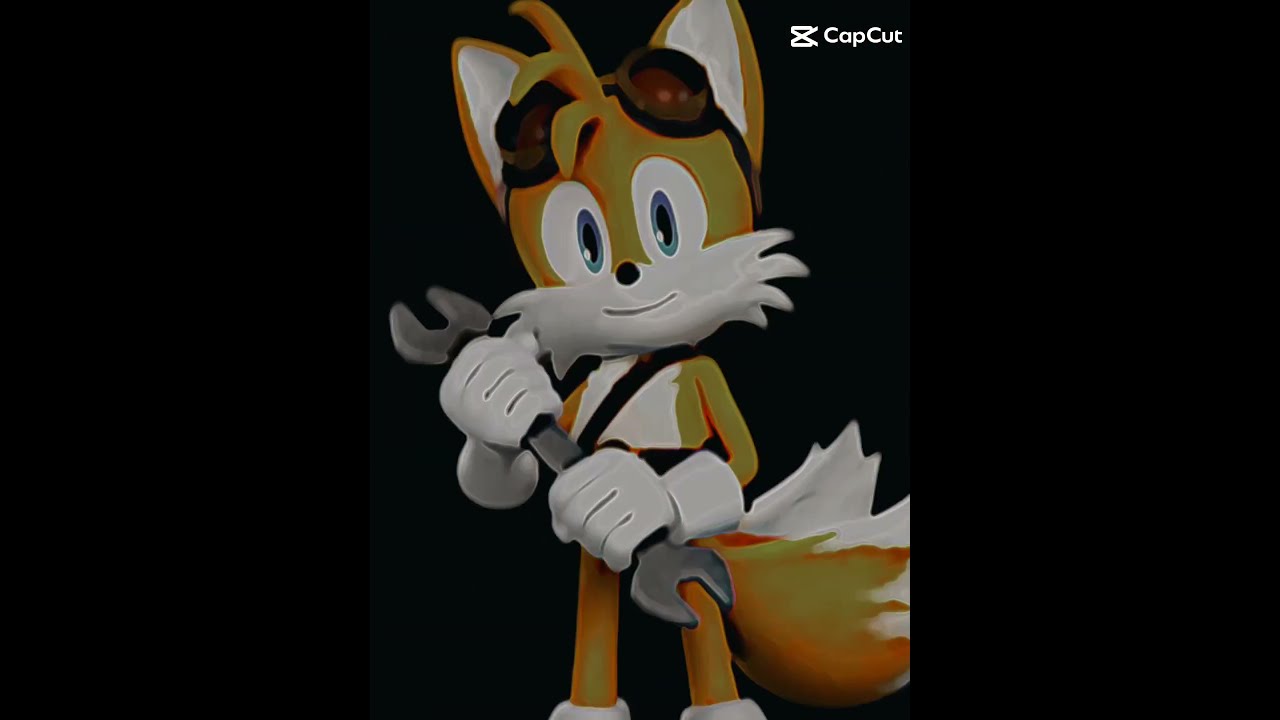The image depicts the famous video game character Miles "Tails" Prower from the Sonic the Hedgehog series by Sega. Tails is an anthropomorphic fox with distinctive twin tails, which he uses to fly. He stands upright on his hind legs, wearing white gloves and white shoes. His fur is primarily a yellowish-orange color, with white fur accentuating his chest, mouth area, and the inside of his ears. Tails has large, expressive blue eyes and a small black nose. On his head, he sports brown aviator goggles situated just above his ears. He is holding a silver wrench in both hands, and a strap akin to a tool belt is visible across his chest. The background of the image is black, and in the upper right-hand corner, the text "CapCut" is displayed. The image is bordered by black rectangles on both the left and right sides.